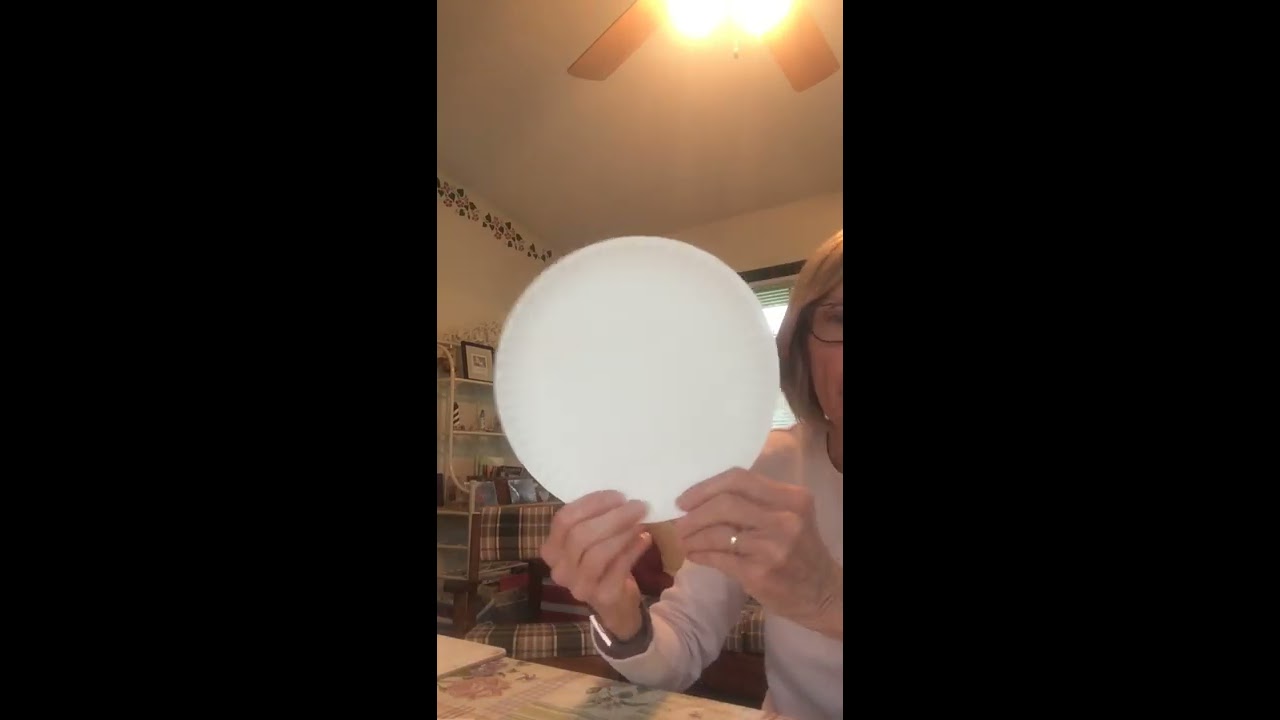In this detailed photograph, a woman, likely in her 50s or 60s with dirty blonde hair, is holding a standard white plate. Partially visible, her face is mostly obscured except for her glasses, which have dark frames, and a glimpse of the right side of her face. She is wearing a beige or light-colored shirt, but her hands are the primary focus of the image. On her left hand, she wears a silver wedding ring and on her right wrist, a wristwatch. She appears to be seated at a table adorned with a tablecloth featuring a pink flower and green leaf pattern. The table has a cutting board and potentially other small items.

The background reveals a cozy, indoor setting with various elements. To her left, the wall is decorated with a floral trim similar in color to the tablecloth. Behind her, a window, likely open as the blinds are pulled up, hints at an airy atmosphere. Above her, a ceiling fan with brown blades and lit yellow lights chirps down, casting a warm glow throughout the room. Further behind, a white shelf holds photographs and assorted baubles, adding to the homey ambiance. Additionally, a plaid chair with dark and white patterns and brown legs is noted among the furniture. The lighting and overall decor suggest a personal and inviting space within her home.